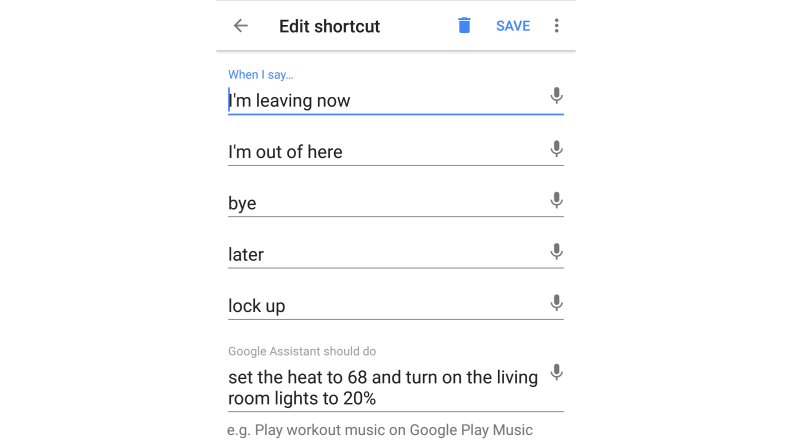In the image, there is a user interface showcasing an edit shortcut feature. The prominent blue "Save" button is accompanied by a trash can icon to its right, followed by a button with three vertical dots, representing additional options. Below, in a smaller blue font, the text reads "When I say:" followed by several command phrases arranged in a vertical list: "I'm leaving now," "I'm out of here," "Bye," "Later," and "Lock up." Each phrase is set to trigger Google Assistant to execute a series of actions: setting the thermostat to 68°F, dimming the living room lights to 20%, and playing workout music on Google Play Music. This setup evidently indicates that, upon saying any of the listed phrases, the Google Assistant will perform the specified tasks to prepare the home for the user's departure.